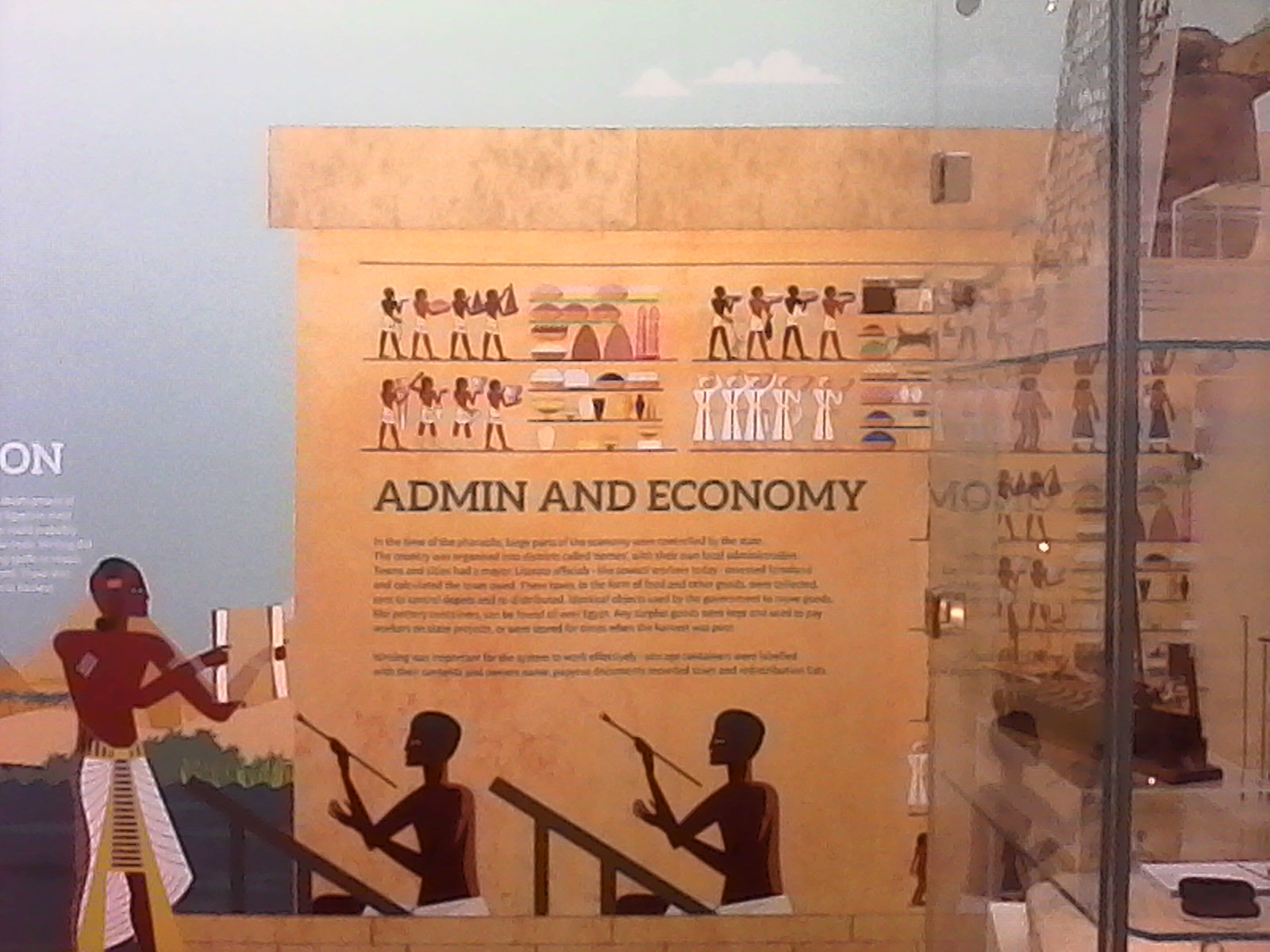The photograph displays a detailed exhibit at a museum focused on Egyptian history, particularly the theme of "Admin and Economy." In the foreground, there is a clear glass case with visible shelves, though the contents are not discernible. Dominating the background is a large drawing set against a brown backdrop, depicting stylized Egyptian figures in traditional poses. Central to this drawing are three Egyptians: one holds a scroll, and two others hold paintbrushes while standing on stairs. Above them, the title "Admin and Economy" is prominently displayed. Beneath this title is a block of black writing and a paragraph that provides additional context, though the text is too small to read clearly. The wall also features two horizontal rows of smaller drawings, each illustrating people engaged in various activities, all rendered in the characteristic Egyptian style. To the right of the drawing stands the clear display case, presumably housing statues or artifacts related to the exhibit’s theme.